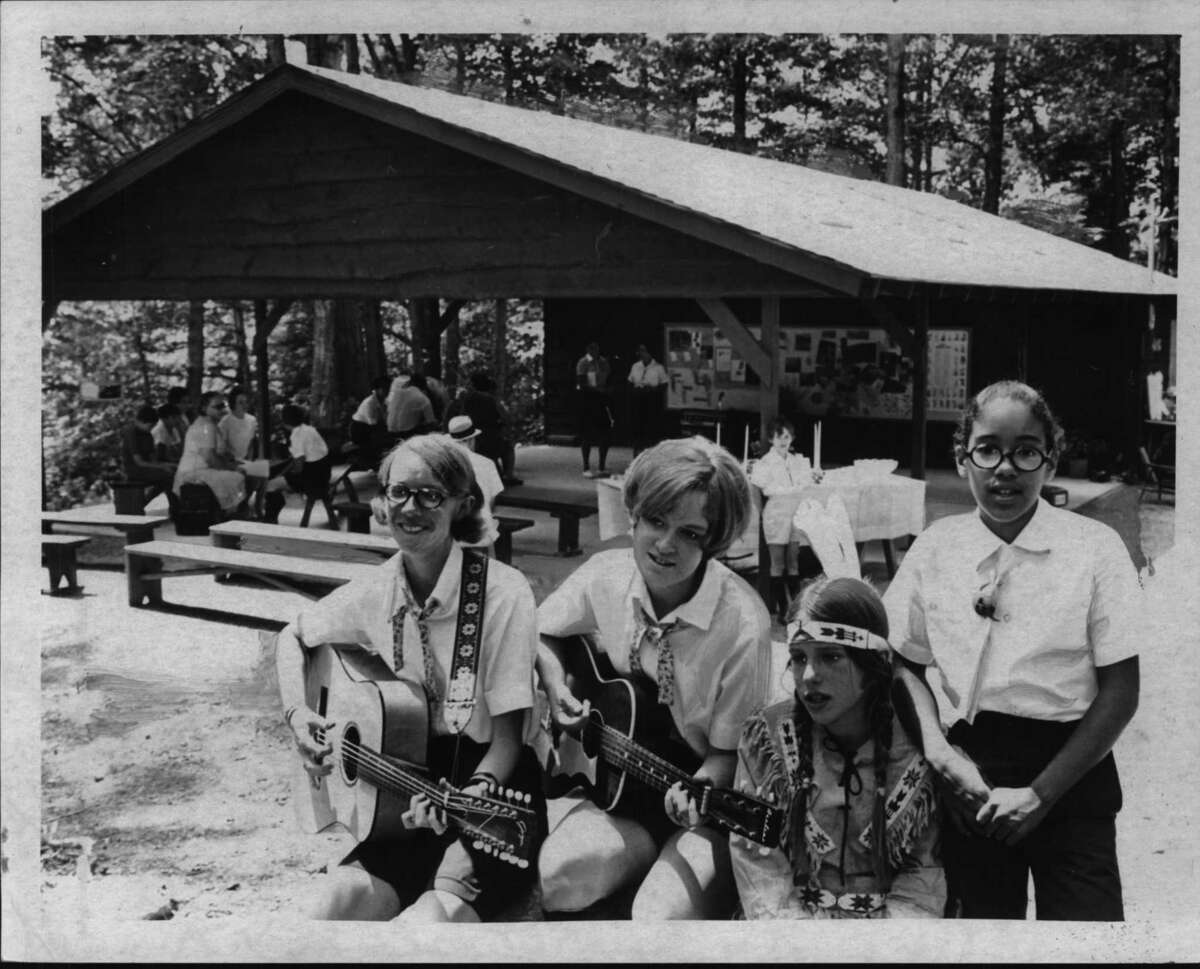This black and white photo, likely taken in the late 60s or early 70s, captures what appears to be a scene from a summer camp set in a forested area. In the forefront, four youth are seated and standing, with two young women playing guitars. Both wear white t-shirts and black pants, resembling a camp uniform. Beside them, a girl dressed in Native American attire with braided hair adds a culturally specific element to the scene. The background features a large, open pavilion with a sturdy roof supported by pillars, housing simple benches and bulletin boards. Several other campers and staff are also visible, some seated on benches beneath the pavilion, which suggests it serves as a communal gathering space. Surrounding the camp, the dense woodland indicates a peaceful, rustic environment.